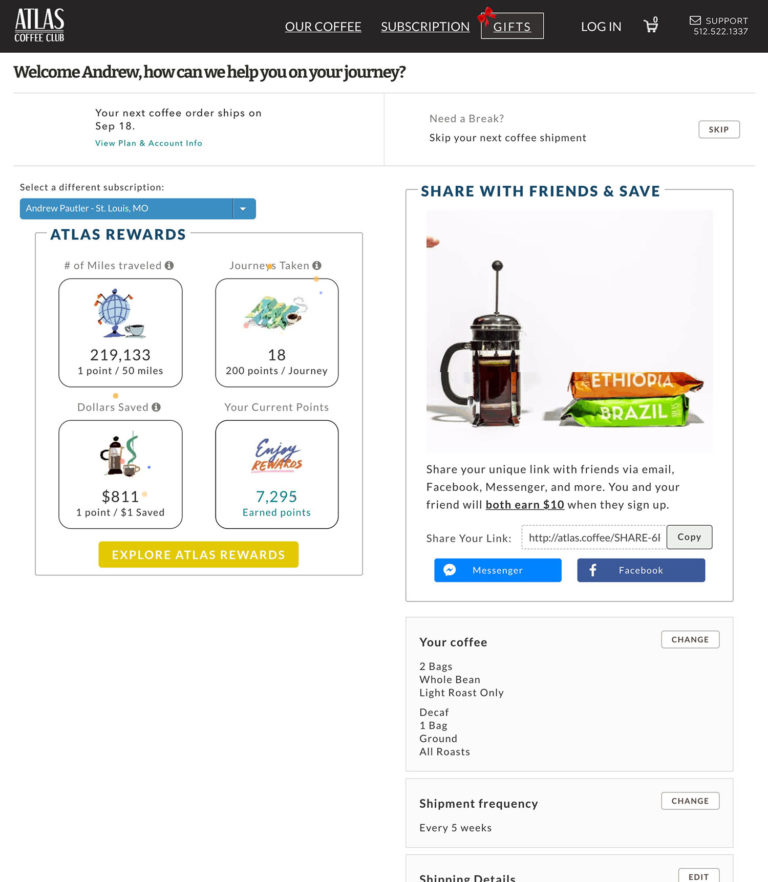A website screen interface featuring the Atlas coffee subscription service is displayed. At the top left corner, the word "Atlas" appears in white text. Adjacent to it, three categories are listed: "Our Coffee," "Subscription," and "Gifts." Further to the right, there is an option marked "Support." 

Beneath the main navigation, the welcome message "Welcome Andrew, how can we help you on your journey?" is prominently displayed. Below this, a rectangular notification reads, "Your next coffee order ships on September 18th" in black and blue text. Smaller text beneath it offers the options "View Plan" and "Account Info." To the right, a message reads, "Need a break? Skip your next coffee shipment" with a "Skip" button nearby.

On the left side, the Atlas Rewards section is divided into four squares: 
- The top left square displays "219,133" travel miles.
- The top right square shows "18 out of 200 points" for journey miles.
- The bottom left square indicates "$811.01" saved.
- The bottom right square presents "7,295" earned points in blue text.

Directly below these squares, a yellow banner reads "Explore Atlas Rewards" in white text, with a "Share with friends and save" option in blue text to the right.

Further down the page, there are images of coffee beans from Ethiopia and Brazil. Beneath these images is a "Copy Link" button that allows you to share via messenger or Facebook.

The order summary at the bottom lists the following:
- Two bags of whole bean, light roast coffee.
- One decaf bag, ground and all roasts.

The shipment frequency and shipping details are displayed at the very bottom of the screen.